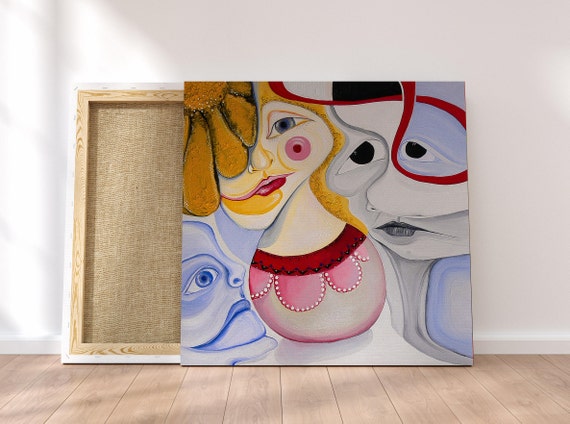In this photograph taken indoors, a modern art painting is prominently displayed, leaning against a white wall with light wooden flooring. To the right, the painting features a series of abstract, melting faces blending into one another, employing a mix of colors such as blue, red, yellow, pink, black, and white. The largest face on the right side boasts a black-and-white palette with detailed eyes and lips, a smeared nose, and rounded lines, reminiscent of a cubist style. Adjacent is a woman's face with orange hair and blue eyes, framed by large orange petals resembling a sunflower, and showcasing big red lips and rosy cheeks. Her body, shaped like a teardrop vase, dons a dress with a red neckline, adorned with pink lace and white dots. To the far left is another woman's face in monochrome blue with exaggerated lips, all blending into this surreal composition. Behind this painting, the back of another brown canvas is visible, adding depth to the scene against the backdrop of white floor molding.